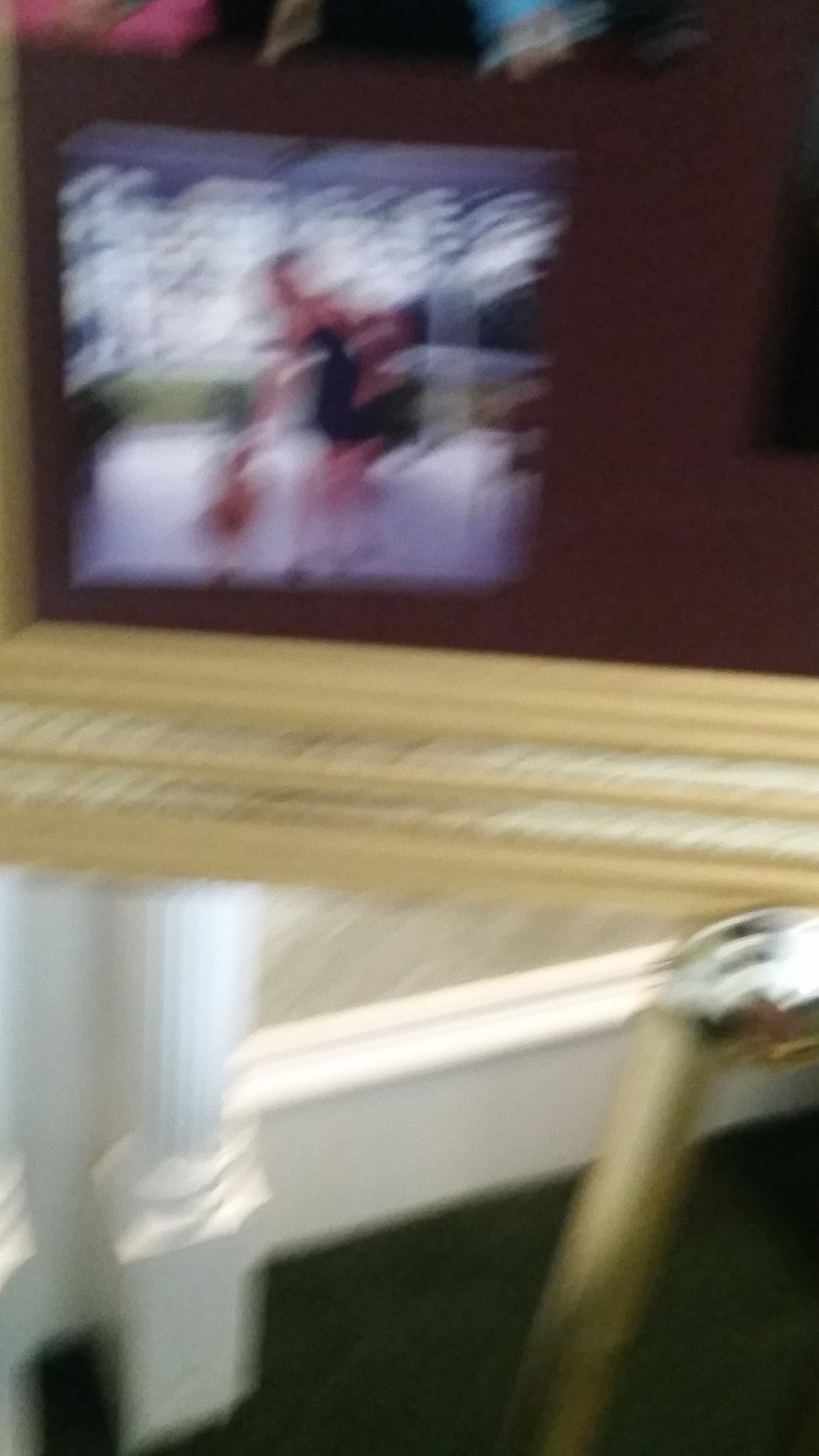In the image, a tall, long, rectangular frame is prominently displayed within a vertical orientation. The frame is an opulent gold with intricate detailing and is set against a rich maroon background. Various pictures, resembling old photographs or small art pieces, are pinned meticulously to this background, creating an engaging visual collage. The frame is supported by a gold easel, enhancing its majestic appearance.

It is evident that this view captures the lower left corner of the display. The setting includes a green carpet that extends from the bottom of the frame towards the baseboard. The baseboard itself is painted white, adding a crisp contrast to the scene. Adjacent to it is the base of a thin pillar, which is square and white, complementing the baseboard. This slender pillar, possibly part of a larger architectural structure, extends upward along the wall. The small segment of the wall visible in the image is adorned with tan-colored wallpaper, adding warmth to the scene.